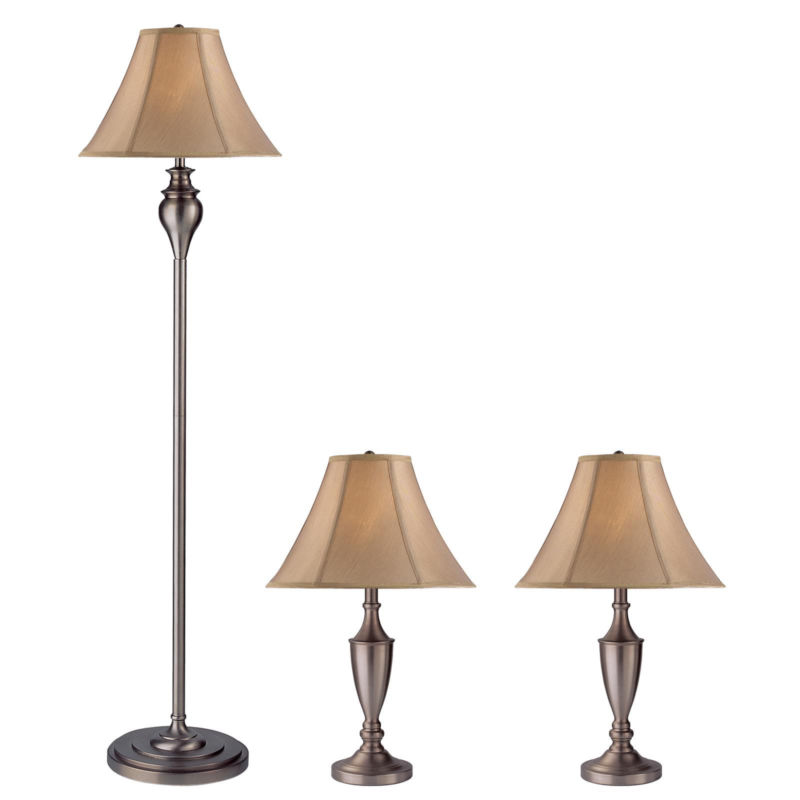In the photograph, three lamps are displayed against a plain white background. To the left, there is a tall floor lamp with a slender, silver-colored metal pole and a base featuring concentric circular rings. The lamp has a vase-like shape just below the flared fabric lampshade, which is a light brown or beige color. Positioned on the right are two matching table lamps, designed similarly to the floor lamp but without the elongated pole. These table lamps have shorter, trophy-like silver bodies with circular bases that taper finely towards their identical beige lampshades. The cohesive design and color palette suggest that all three lamps are part of the same collection, ideal for creating a harmonious lighting setup in a living space.